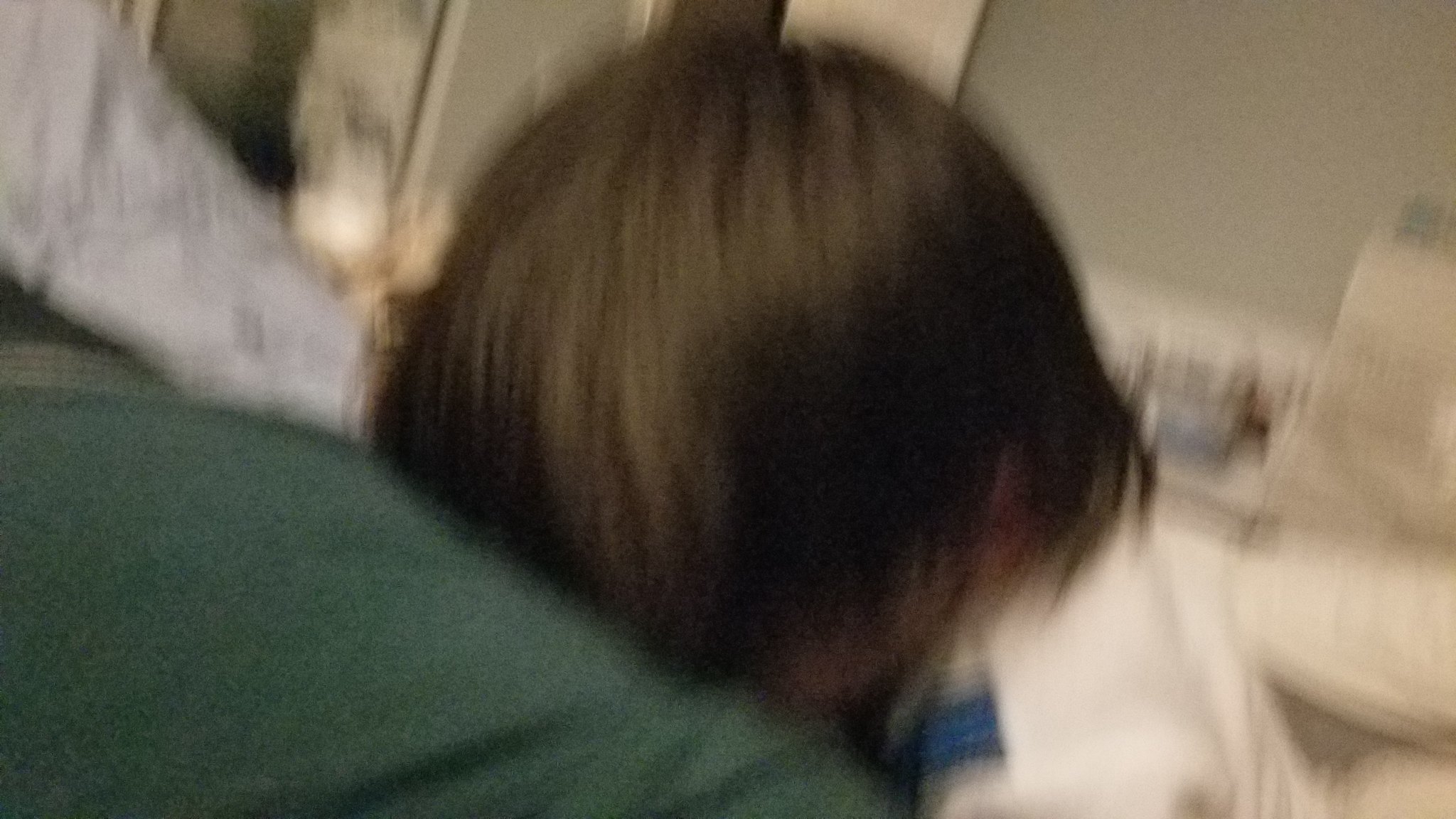The image, although mostly blurry, centers on the top of a person's head, showcasing their long, straight, silky, dark brown hair that falls just to their shoulders. The person's shoulders, bathed in white, are visible to the right of the image, suggesting they might be bowing their head downwards into a green blanket positioned in the lower left corner. A white pillow rests on this green blanket in the upper left part of the photo, adjacent to a rectangular light or lamp. To the right, the photo reveals what seems to resemble a bathroom counter, complemented by light gray walls. Beneath the counter, a silver tray holds various items, completing the scene.